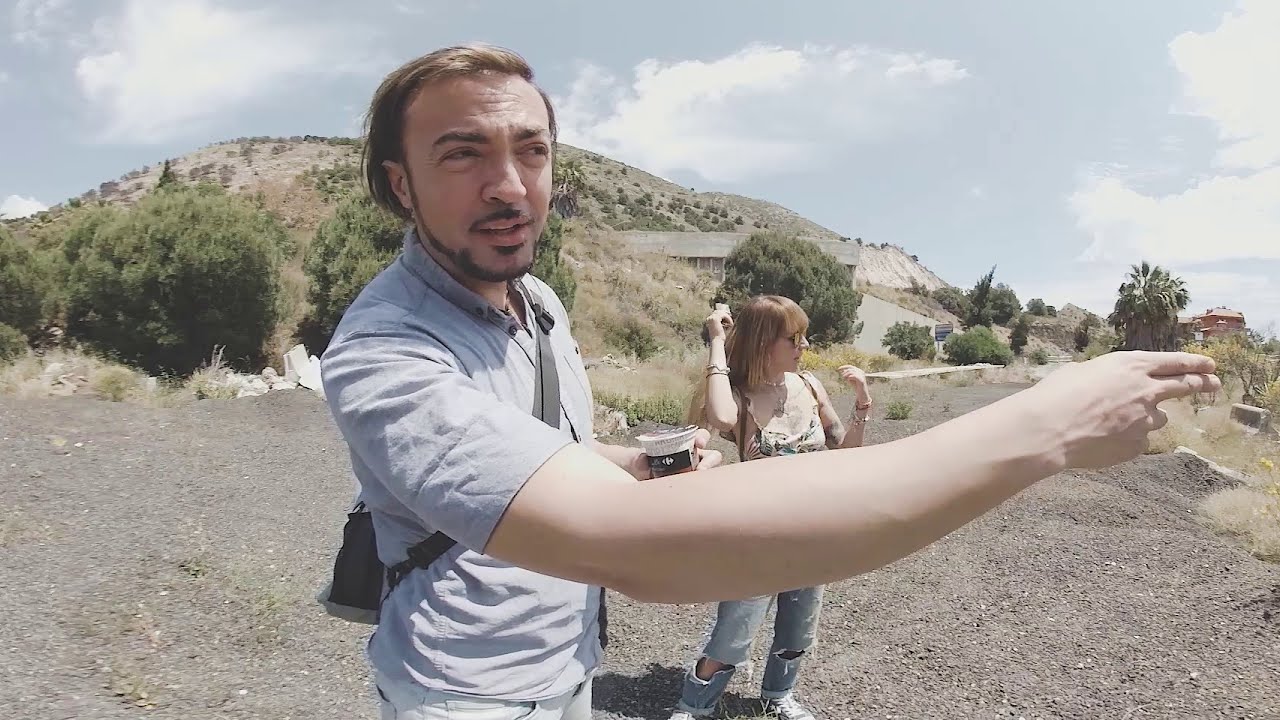In this outdoor photograph taken near the top of a mountain or foothill, a man with a closely cropped beard along his jawline and a thin mustache, receding brown hair combed back to his collar, stands prominently in the foreground. He is dressed in a short-sleeved gray (or light blue) button-up shirt and has a cross-body bag strap over his shoulder. The man, who appears to be holding a beverage, is pointing to the right of the image with his right hand, and his arm looks unusually large due to the perspective. Behind him is a woman with shoulder-length brown hair, glasses, and bangs, wearing a sleeveless patterned top and ripped jeans with sneakers, and bracelets on both wrists. She is also looking to the right, possibly combing her hair. They stand on a wide expanse of gray gravel, with a small hill in the background, featuring scattered bushes, scrubby foliage, and perhaps some lower palm-type plants. The sky is pale blue with fluffy white clouds, suggesting a clear, daytime setting in a drier, arid climate. Some buildings or homes are faintly visible off to the right in the distance.